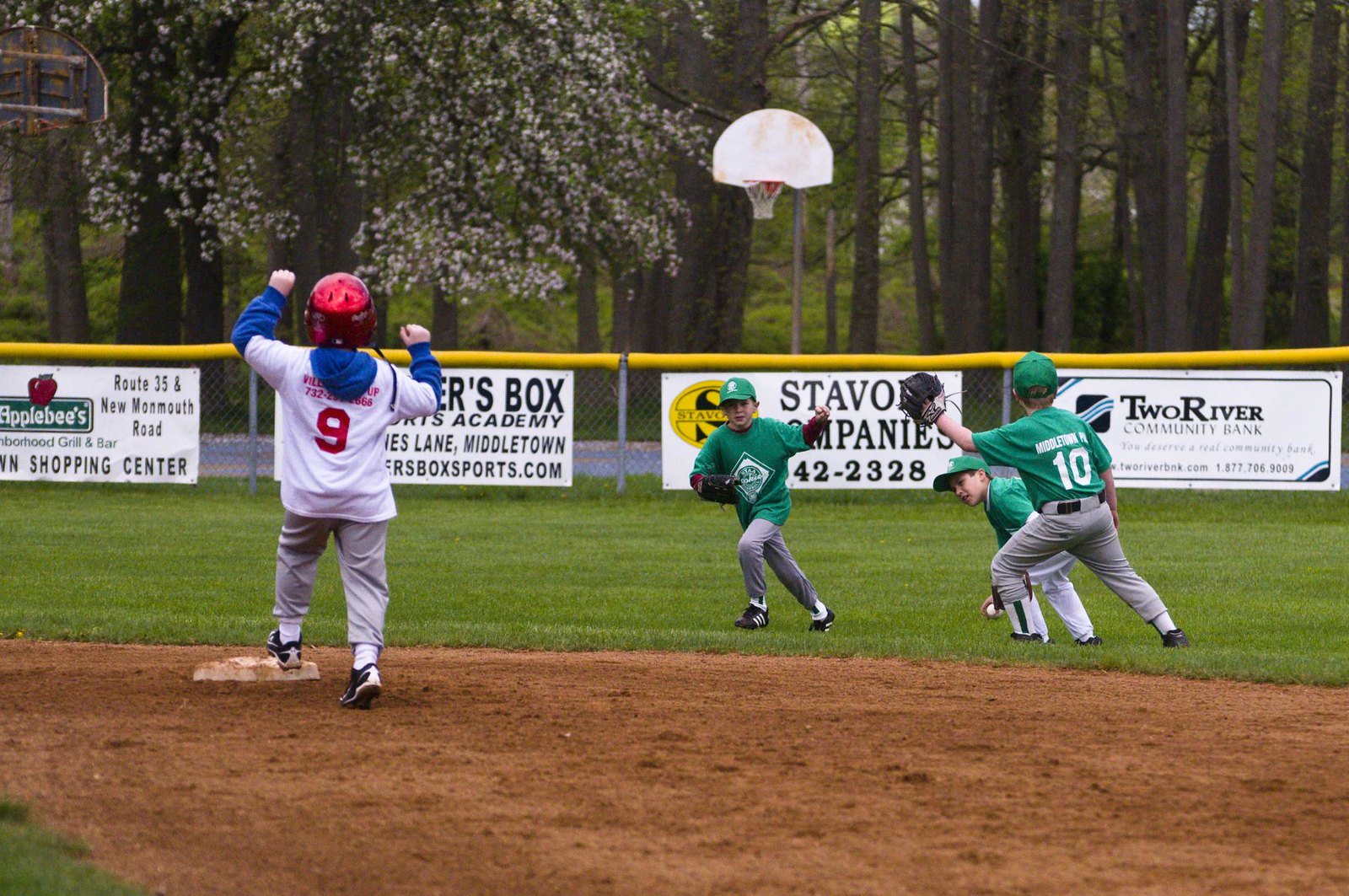This photograph captures a lively outdoor scene at a children's little league baseball game. In the foreground, a child in a white jersey with gray pants and a red helmet stands on a base, having just secured his position. His uniform overlays a blue hoodie, with a red number nine on his back. To his right, three other boys in green jerseys with gray pants are actively engaged in the game. One boy with the number 10 on his back is positioned with his catcher's mitt extended, facing away. Another is bent down picking up a ball, while the third is running toward the pitcher's mound. 

The baseball diamond's brown dirt stands in contrast to the surrounding green field. Behind the players, a chain-link fence with a yellow protective barrier lines the field. Attached to the fence are various advertisements, including banners for Applebee's, a shopping center, an academy, and the Two River Community Bank. Beyond the field, tall trees create a lush backdrop, which includes a flowering white tree. Additionally, a white backboard basketball hoop is visible, hinting at another sports area nearby. The scene is filled with activity and the essence of a vibrant community event.